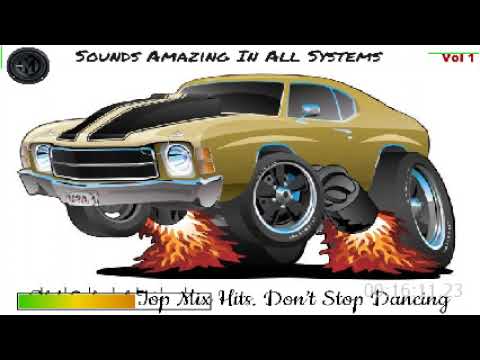The image features a detailed, artistic depiction of a golden muscle car facing left and slightly forward, accentuating its powerful design. The car exhibits a prominent black stripe down the middle of the hood, highlighted by white detailing. Notably, its left rear tire appears angled, reminiscent of an action-packed scene, and the front tire seems to be airborne. Enhancing its dynamic appearance, large orange flames burst from cannons protruding below the driver's door and the right-hand side, giving the impression that the car is being lifted off the ground. The background is stark white, accentuating the car and making it stand out vividly. The image is framed with thick black borders at the top and bottom. At the top, bold black letters proclaim, "Sounds amazing in all systems," accompanied by "VOL1" on the right and a circular design on the left. Below the car, partially obscured by a green and gold bar, the text reads, "Top mix hits. Don't stop dancing," suggesting a lively and energetic theme. This detailed and animated illustration could well be an album cover, blending elements of retro and modern design.